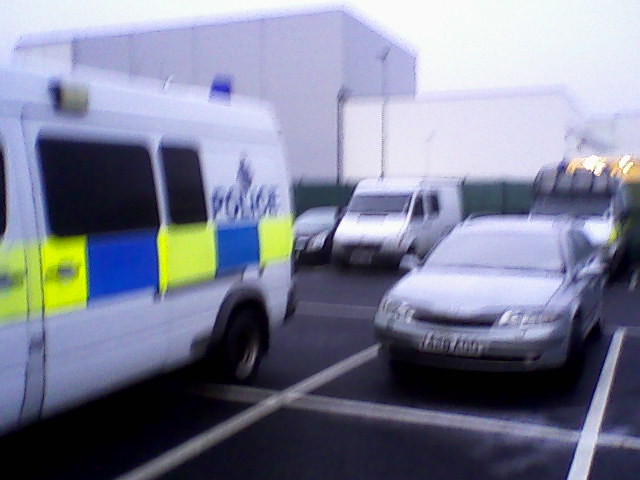This is a very blurry photograph of a parking lot featuring several cars and a prominent police van. The parking lot has black pavement with white lines marking the parking spaces. In the foreground, on the right side, there is a silver car with a blurred-out license plate and small roof bars, parked adjacent to a white delivery van with cargo on its top. To the left, there's another white van with tinted windows and a word "police" written in dark blue, accompanied by yellow and blue checkered squares along its sides. The background reveals industrial-looking buildings: a large gray square building next to a smaller white one, separated from the parking area by a dark green wall. Various other parked vehicles include a black coupe. The police van partially visible on the left has distinctive black windows and an alternating yellow and blue striped band across its side, further marked by the word "police" in blue text on a white background. This photograph might depict a police station's parking area, suggested by the presence of the police van and industrial buildings in the background.